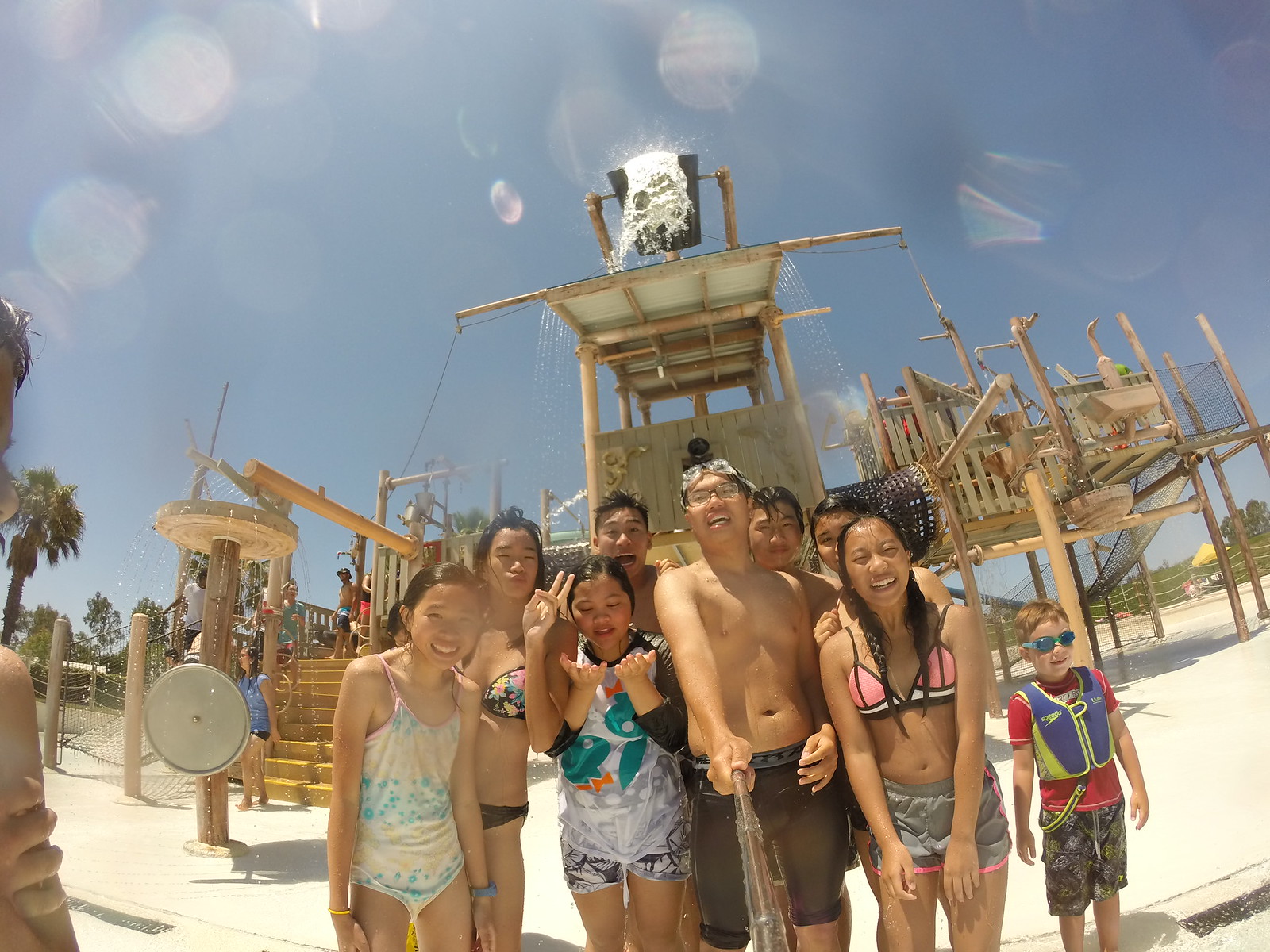In the photograph, a cheerful group of around eight kids of various ages, including both boys and girls, are standing in front of an elaborate, hand-built wooden climbing structure on a beach. This structure features multiple nets, suspension bridges, and slides, reminiscent of a treehouse-style jungle gym. A bright, sunny day enhances the scene, with reflections of sunlight visible at the top of the photo. The kids, all dressed in swimwear and some wearing life jackets, appear to range in age from approximately six to fourteen years old. They are accompanied by a man and a woman, likely in their 30s, who may be their parents. The man is taking the picture with a selfie stick. The structure behind them has a large water bucket at the top, which is seen pouring water, adding a splash pad element to the beach setting. Everyone is laughing and smiling, clearly enjoying a fun-filled family outing.